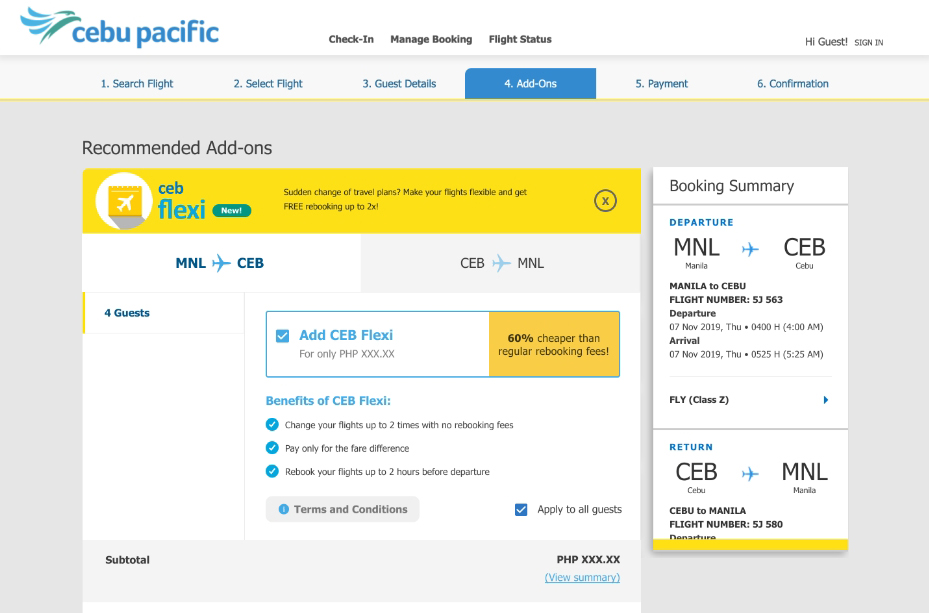The image depicts a screenshot of a computer desktop displaying a webpage from Cebu Pacific's website. At the top left corner, the Cebu Pacific logo is prominently featured in blue text. Centrally, three options are visible in black text: "Check-in," "Manage Booking," and "Flight Status." On the top right, the site welcomes the user with "Hi Guest, Sign in," also in black text.

Below these elements is a white navigation bar with several options sequentially listed: "Search Flights," "Select Flights," "Guest Details," "Add-ons," "Payment," and "Confirmation." These options, except for "Add-ons," are highlighted against a blue background and are written in white text. The "Add-ons" option stands out with a blue background, and above the navigation bar, the text "Recommended Add-ons" is displayed.

There is also a pop-up element featuring a yellow background band with text—mostly in blue, with some sections in black. This pop-up contains additional information or prompts related to the navigation process within the website.